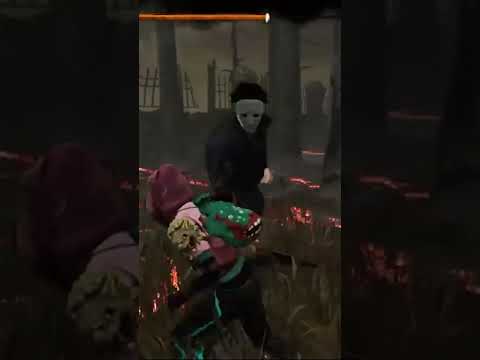The image appears to be a low-resolution, pixelated screenshot from a dark, cemetery-themed video game, possibly resembling a "Fortnite" setting but with a spookier, nighttime ambiance. The scene is divided into three parts: a central main picture flanked by two darker, zoomed-in sections of the same image on the sides. The central image depicts a young woman in a red hoodie, pink top, black pants, and a green backpack adorned with a mouth featuring red lips and jagged teeth. She is seen running through foliage and what seems to be flaming grass, away from a menacing figure. This figure, dressed in a dark jumpsuit and a white mask, closely resembles Michael Myers from the Halloween series. The backdrop shows broken cast-iron fences, scattered tombstones, and towering pillars typical of old cemeteries, while a dark wooded area looms in the distance. A partially visible health meter at the top suggests gameplay elements.